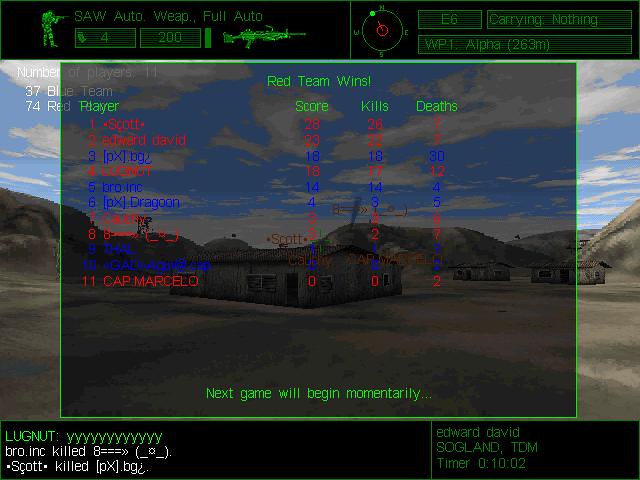This image captures a paused moment in a shooting video game, likely viewed on a computer screen. The main scene is a digitally rendered desert valley, featuring rugged rocky mounds and barren, tan ground punctuated by three simple, rectangular, single-story buildings. The background showcases a vibrant sky with scattered clouds overhead. 

Overlaying the game scene, a semi-transparent gray pop-up announces in green text that the "Next game will begin momentarily", with "Red Team Wins" prominently displayed. Red and blue text tally the scores, kills, and deaths for each team. Black bars along the top and bottom of the screen contain various in-game information. 

The top bar shows a green silhouette of a military figure holding a gun, accompanied by icons indicating the player's weapon status (described as a "SAW auto" or "full auto" gun) and a compass showing their direction—facing nearly north with a slight westward angle. Additional data such as health and weapon power bars, and rectangular detail tabs, provide more player stats.

The bottom black bar includes details of recent kill counts, mentioning players like "lug nut bro, ink killed eight" and "Scott killed p x b g". This detailed overlay offers a comprehensive view of the player's status and the game's progression at the paused moment.